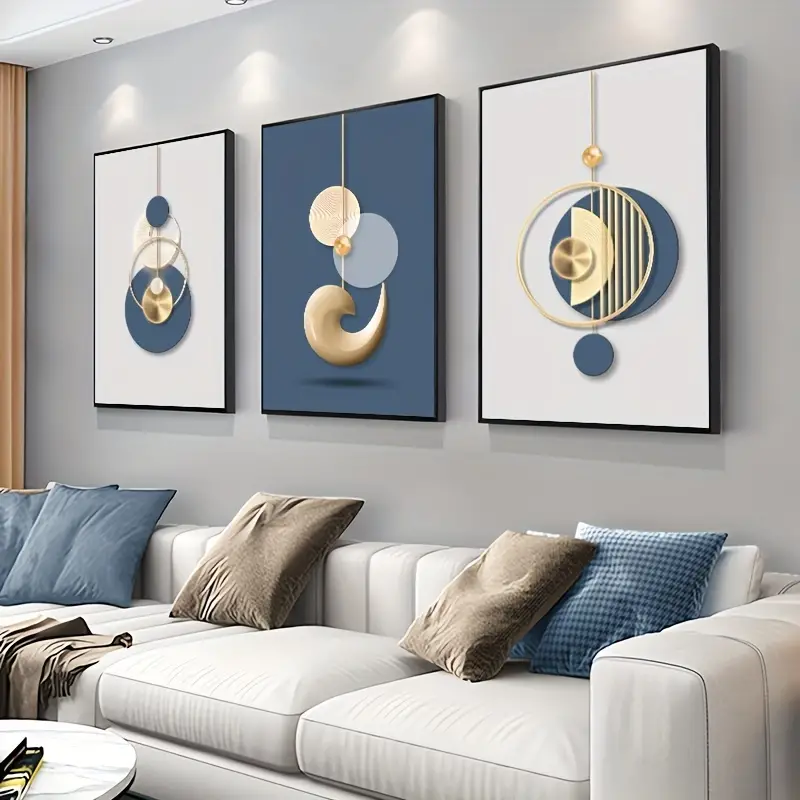This image showcases a stylish living room with light gray walls adorned by three contemporary art pieces. Each artwork features intricate designs of circles and other geometric shapes, incorporating a consistent color scheme of light blue-gray, dark blue-gray, gold, and tan. The paintings are similar in style, with variations in the arrangement of the shapes; the left and right pieces have white backgrounds, while the center piece has a dark blue one, all hanging under a soft glow projected by ceiling-mounted halogen lights.

Below the artwork is a long, light gray sofa accented by dark blue-gray and dark tan pillows, as well as a wrinkled, dark tan blanket partially draped over its edge. The room also includes a circular, white table, enhancing the modern and cohesive aesthetic of the space.